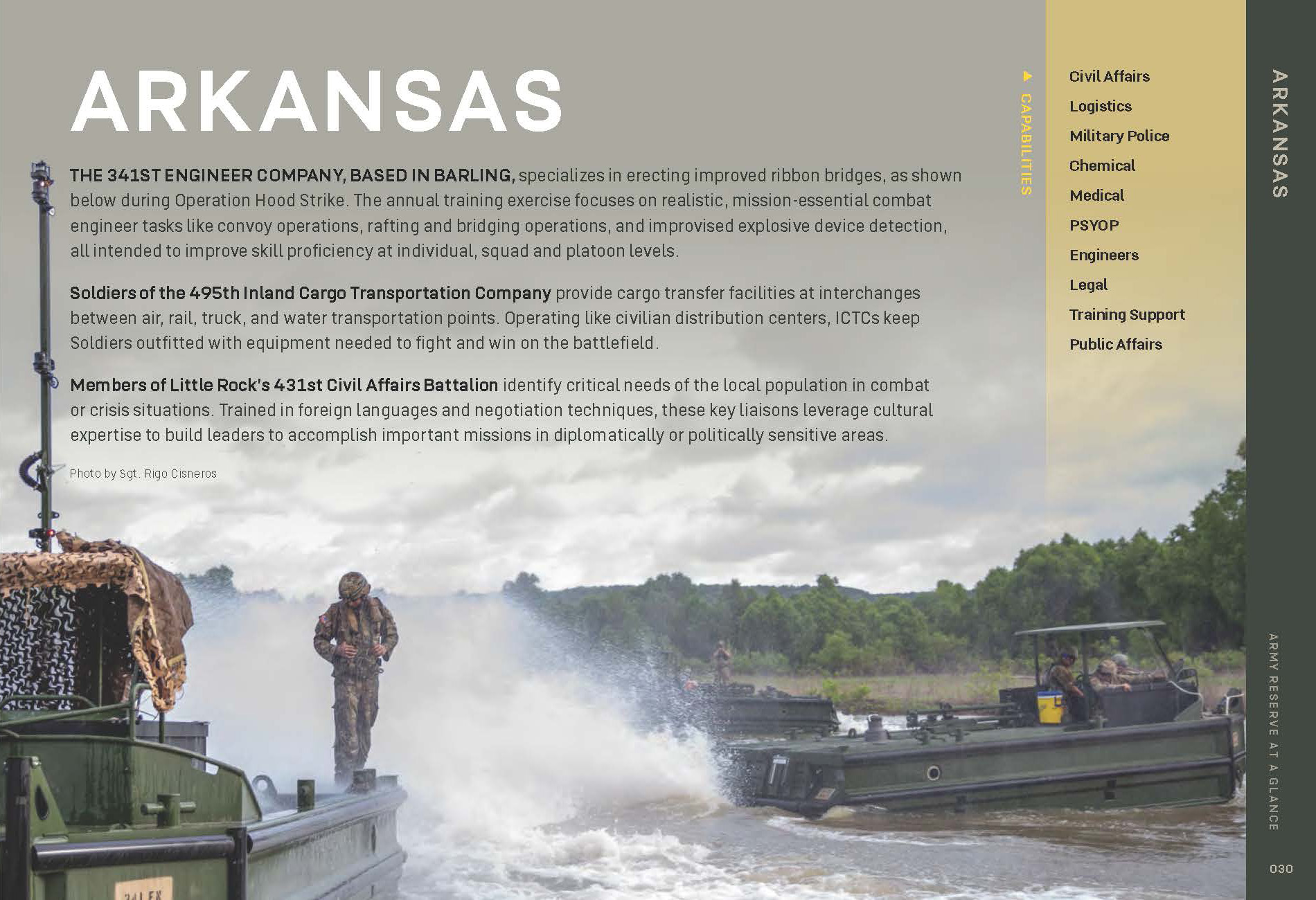The image depicts a detailed scene from the state of Arkansas, presented in a layout reminiscent of a page from a book or a PowerPoint slide, possibly a poster. At the top, the title "Arkansas" is prominently displayed in white lettering. Below the title, there are three sections of text providing an overview of various military operations and units based in Arkansas. The first section details the 341st Engineer Company from Barling, which specializes in erecting improved ribbon bridges during exercises like Operation Hood Strike, focusing on essential combat engineer tasks. The second part describes the role of the 495th Inland Cargo Transportation Company, which handles cargo transfers between different transportation points, similar to civilian distribution centers. The third section highlights the 431st Civil Affairs Battalion based in Little Rock, which identifies local needs in crisis situations, leveraging language and negotiation skills for sensitive missions.

Below these descriptions, a vivid image captures a soldier dressed in camouflage fatigues and a helmet, standing on the edge of a boat. To his right, there are two army green boats; one appears to be stationary, facing the camera, while the other is moving, kicking up water behind it. Each boat carries soldiers, with three in one and two in the other. The background features green trees and hills under a cloudy sky, and the overall scene is filled with earthy tones, suggesting a river or swamp setting with muddy water.